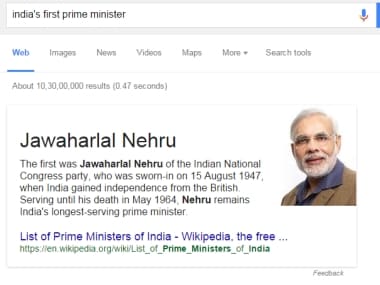This screenshot captures a detailed Google search result for India’s first Prime Minister. Set against a white background, the search interface prominently features a search bar at the top where the query "India's first prime minister" has been entered. Adjacent to the search bar on the right is a blue microphone icon. Below the search bar, navigation tabs allow users to filter the results by category, with options labeled 'Web' (highlighted in blue and underlined, indicating it has been selected), 'Images,' 'News,' 'Videos,' 'Maps,' 'More' with a dropdown menu, and 'Search tools.'

The search yields approximately 10,030,300 results in 0.47 seconds, as accurately detailed beneath the navigation tabs. The central part of the screenshot showcases a knowledge panel box featuring a photograph of Jawaharlal Nehru, the first Prime Minister of India. Nehru is depicted wearing a brown suit with a blue shirt, glasses, and sporting a white beard, mustache, and hair. He has brown eyes and an Indian heritage. 

To the left of his photographic image, the text provides a concise biography: "Jawaharlal Nehru, a key figure in the Indian National Congress Party, was sworn in on August 15, 1947, when India gained independence from British rule. Nehru served as Prime Minister until his death in May 1964, making him India's longest-serving Prime Minister." 

At the bottom of this section, a blue hyperlink directs users to a more comprehensive list, titled “List of Prime Ministers of India - Wikipedia, the free.” Below this link, the website URL is displayed in green: "https://en.wikipedia.org/wiki/List_of_Prime_Ministers_of_India." Finally, in the bottom right corner, the word "Feedback" appears in grey font, inviting users to provide input on their search experience.